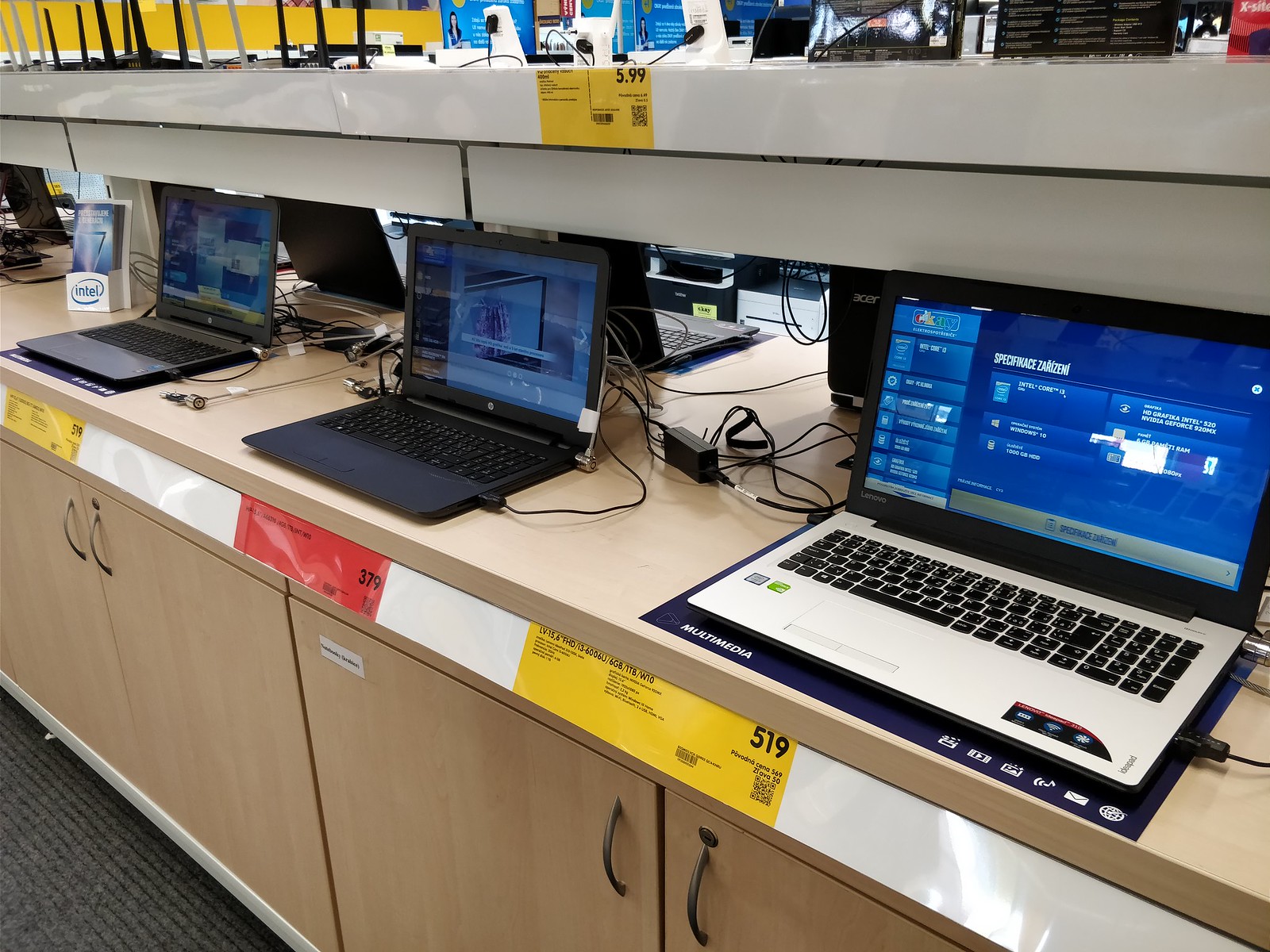The photograph captures an interior scene from an electronics store, prominently featuring a beige-colored display countertop with closed double-door cabinets beneath. The countertop is aligned from the lower right to the upper left and has three open, lit-up laptops neatly positioned in a row. The rightmost laptop appears larger with a white surface surrounding black keys, while the other two laptops are black and smaller in width. Each laptop is accompanied by a detailed spec sheet affixed to the edge of the countertop, right below them. The label for the laptop in the foreground shows the number 519 on a yellow piece of paper, the middle one displays 379 on a red piece of paper, and the label for the backmost laptop also has a yellow paper, although its number and specifics are not fully visible. In the upper left corner of the image, there's a small card holder with a white pamphlet marked "Intel." The setting suggests a typical layout possibly found at an office supply store like Staples, with additional shelves above the countertop, some visible wires, and gray carpeting on the floor.